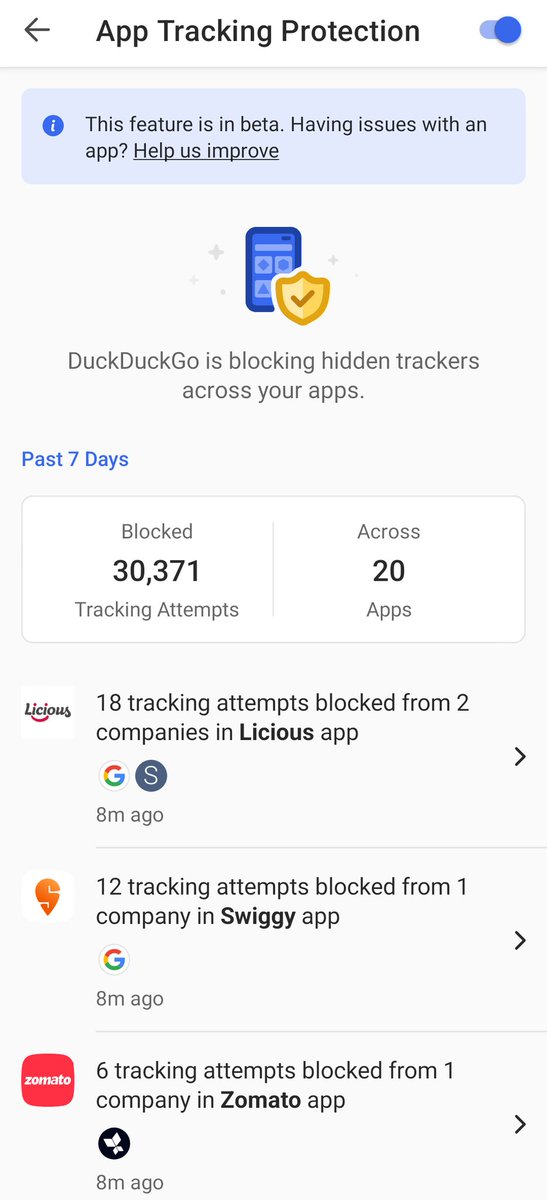**Detailed Caption for Screenshot:**

This image captures a screenshot from a user's phone displaying the settings for DuckDuckGo's App Tracking Protection feature. The background is predominantly white. At the very top, there is a back arrow pointing to the left followed by the heading "App Tracking Protection," indicating that this feature has been activated. The toggle switch is blue, signifying that it is turned on. 

Below the toggle, there is a light blue bar with text inside stating, "This feature is in beta. Having issues with an app? Help us improve," suggesting this is interactive and could be a clickable link for user feedback.

The central part of the screen shows an illustration: a blue smartphone with a yellow shield superimposed on it, featuring a check mark in the shield, symbolizing security and protection. Directly below the image, it reads "DuckDuckGo is blocking hidden trackers across your apps."

The next section includes a time frame option labeled "Past seven days" in blue, with two statistics boxes underneath. The first box states, "Blocked 30,371 tracking attempts," while the second one notes, "Across 20 apps."

Beneath these statistics, there are three detailed entries about specific tracking blocks:
1. A section indicates 18 tracking attempts blocked from two companies within the "Licious" app, featuring the Licious app banner on the left.
2. The next entry shows 12 tracking attempts blocked from one company in the "Swiggy" app, accompanied by the Swiggy logo.
3. Lastly, there is an entry for the "Zomato" app, showing six tracking attempts blocked from one company, along with the Zomato app icon.

The time stamps for the Swiggy and Zomato app blocks both read "eight minutes ago," marking recent activity.